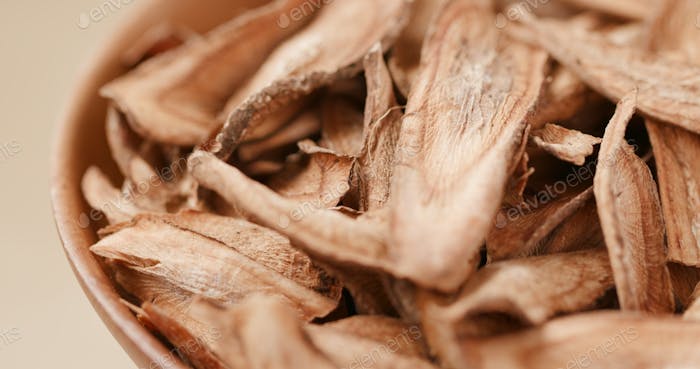The image features an extreme close-up of a tan to brown wooden bowl containing various thin, dry, natural objects that resemble either wood chips, dried mushrooms, or thinly sliced tree bark. The contents are light beige with a rough, textured appearance and craggedy brown or grayish edges, featuring natural ring patterns that suggest they might be part of a plant. The bowl sits against a tan or beige background. Faint white writing is visible on or over the contents, with discernible letters "E-N-V-A-T-O-E" and a partial "E-N." The overall scene has an earthy, organic look with a warm, light tone emphasized by a source of light illuminating the objects.